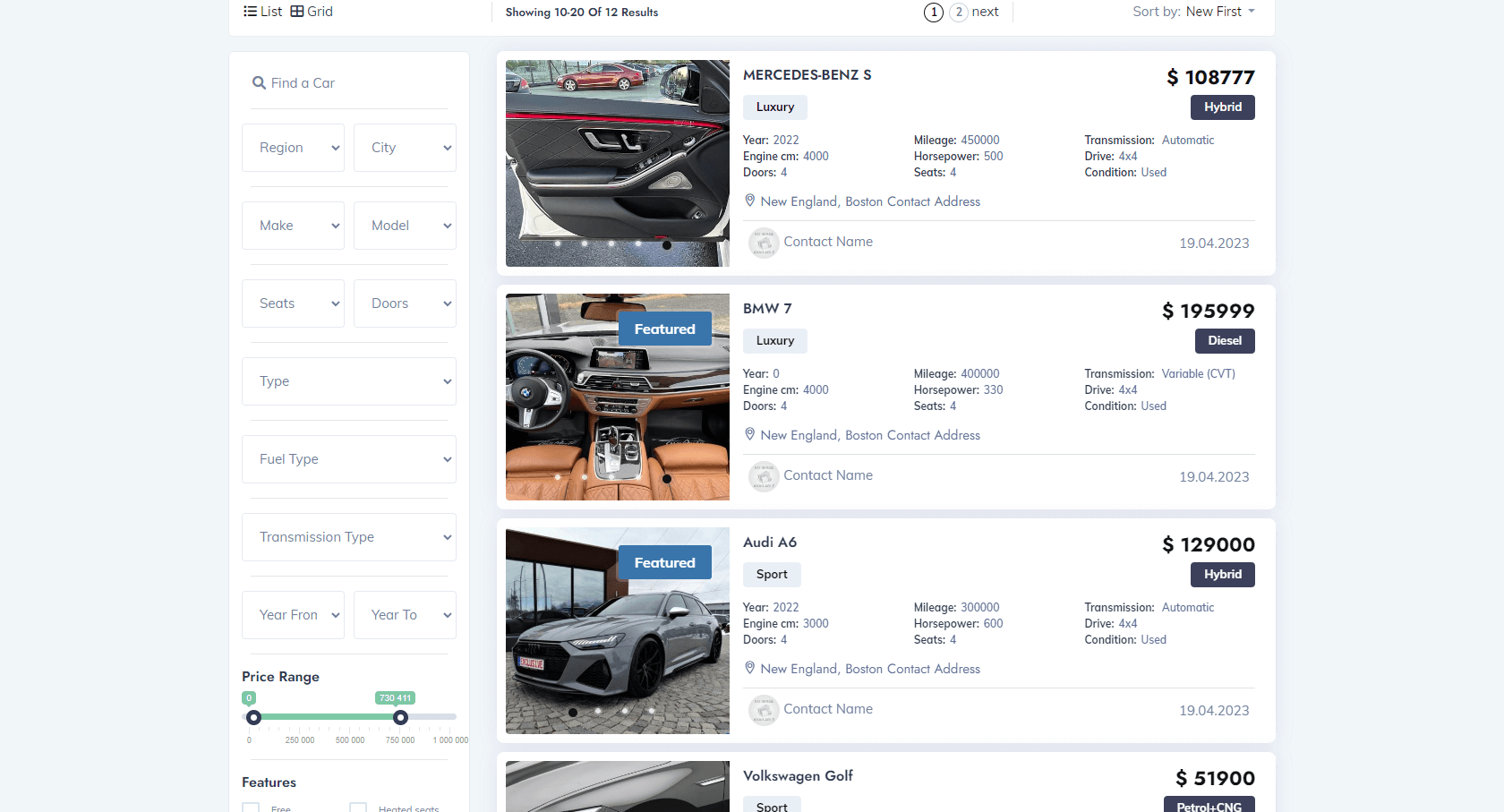Screenshot of an online search interface for luxury cars displayed in a list format. The top of the interface includes a navigation bar with options to toggle between list and grid views. The list view shows a range of vehicles, indicating results 10 to 20 out of 12 brands. A drop-down menu allows sorting by criteria, currently set to "Sort by: New First."

Below this, the search functionality is quite detailed, providing filters for region, city, make, model, number of seats, number of doors, car type, fuel type, transmission type, year range, and price range. In the current search, only the price range filter has been applied.

Four cars are displayed:
1. **Mercedes-Benz S**: A luxury vehicle priced at $108,777, highlighted by an interior shot of the car door.
2. **BMW 7 Series**: An opulent model priced at $195,999. 
3. **Audi A6**: Priced at $129,000, with an exterior shot emphasizing its sleek gray finish.
4. **Volkswagen Golf**: Priced distinctly lower at $51,900, it stands out as the more economical choice within this luxury lineup.